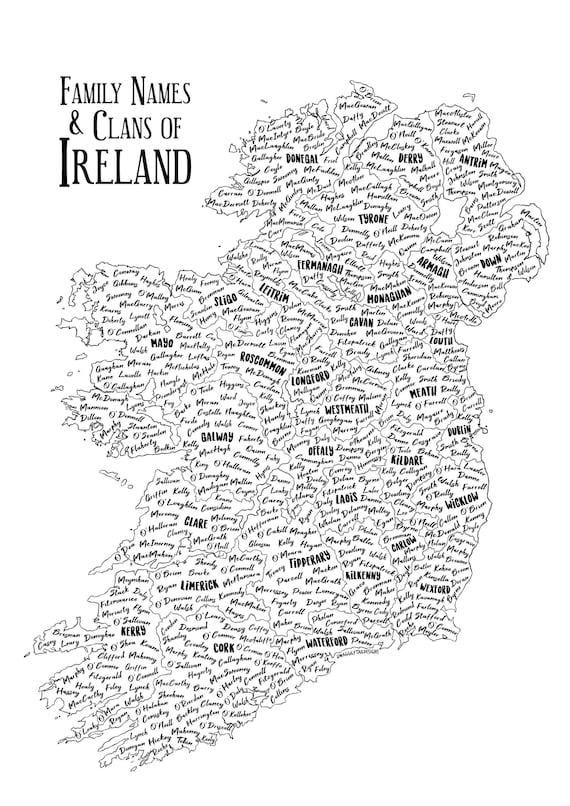This black and white map titled "Family Names and Clans of Ireland" showcases Ireland divided into its counties, with each county's name prominently displayed in bold, capital letters. Surrounding these larger county names, the map is densely populated with thousands of smaller family names and clans written in cursive script. The map's accurate geographical outline of Ireland includes regions such as Cork, Donegal, Derry, Antrim, Tyrone, Down, Cavan, Westmeath, Kildare, Wicklow, Limerick, Kerry, Waterford, Galway, Mayo, Sligo, Roscommon, Longford, Offaly, Kilkenny, Carlow, and Wexford. Each county encompasses a multitude of surnames, creating an intricate and detailed representation of the historical and familial divisions within Ireland.